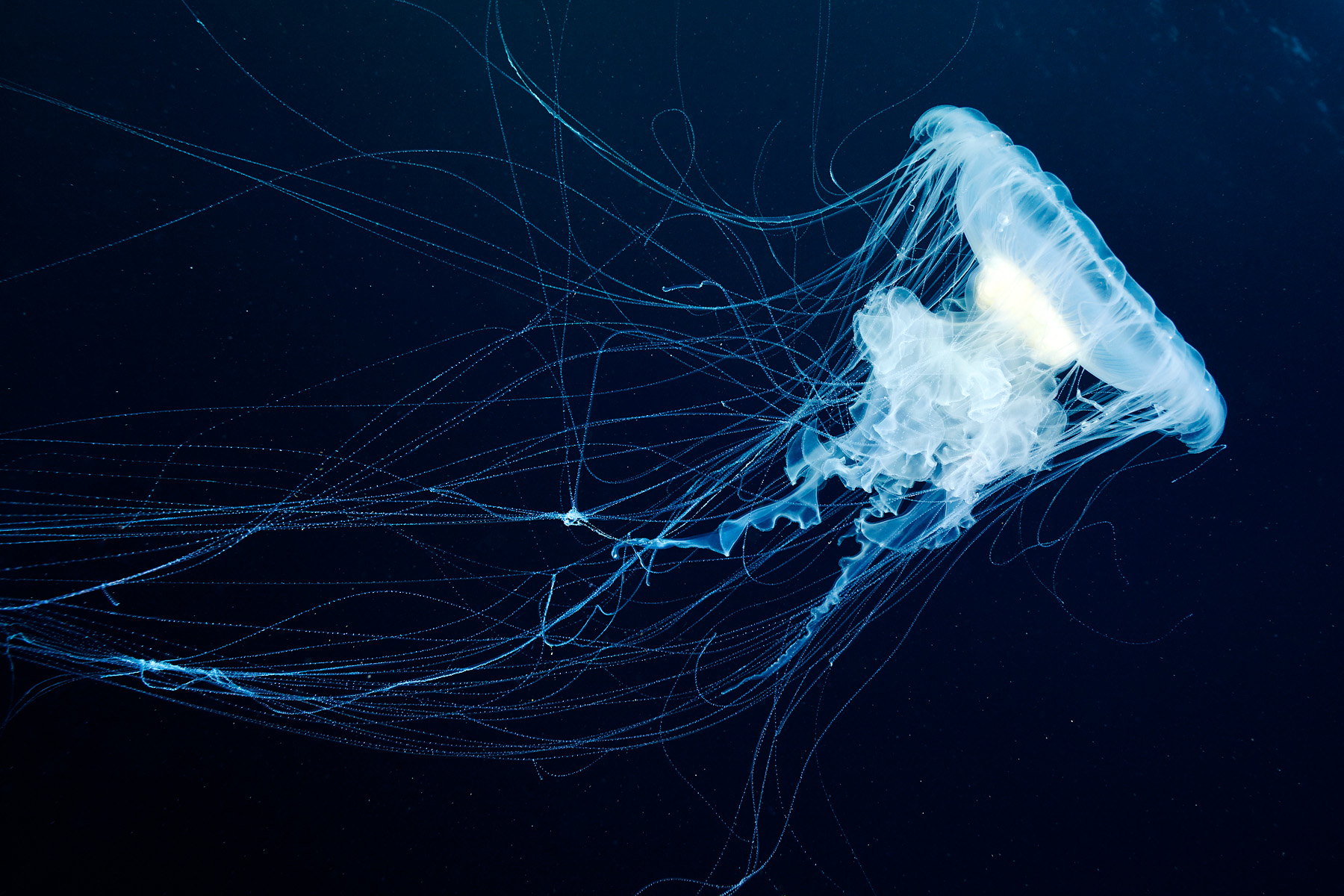This captivating image features a mesmerizing jellyfish, which dominates approximately three-quarters of the frame. The jellyfish is positioned at an intriguing angle, with its ethereal tentacles extending from the center-right edge of the photograph. These long, wispy strands, reminiscent of electrified strings, spread across the right side and middle of the image, adding a dynamic elegance to the scene.

The jellyfish's body is situated almost entirely on the left side of the picture, swooping upward toward the top-left corner in a graceful arc. The scene is set against a dark, deep blue backdrop, enhanced by striking neon blue and electric blue highlights that accentuate the jellyfish's translucent form. 

The central portion of the jellyfish resembles soft, fluffy clouds or cotton candy, creating a stunning contrast with its luminous, flat bell-shaped top. This part of the jellyfish glows with a vibrant electric blue hue, adding to the dramatic and breathtaking visual impact of the image.